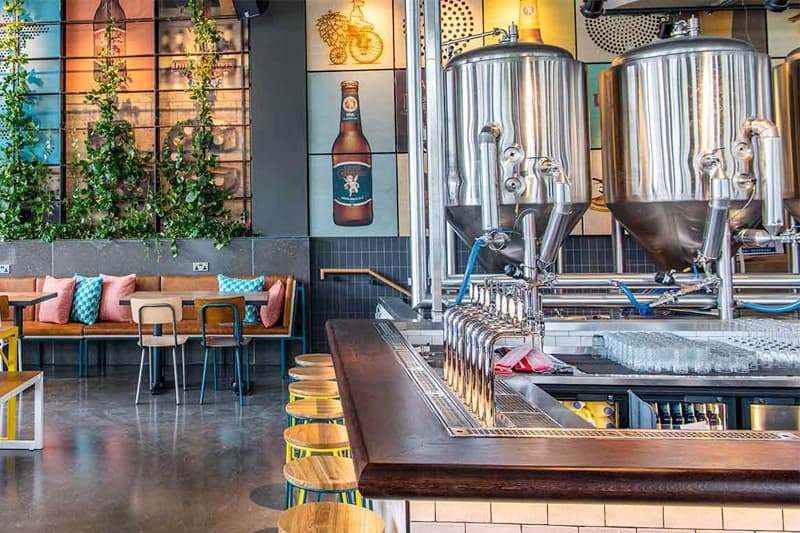This photograph captures the interior of a modern, hip microbrewery with a distinctive blend of indoor and outdoor flair. The central feature is a large, L-shaped wooden bar with lighter wood stools that have yellow and blue legs, creating a vibrant contrast. This bar, adorned with tiles underneath and shiny flooring all around, is where patrons can watch the brewing process and enjoy freshly made beer from the numerous dispensers. 

To the right of the bar are sizable vats with tubes, indicative of the on-site brewing operation. The bar area is further accentuated with large, eye-catching pieces of artwork, including depictions of a wine bottle, a beer bottle, and a cyclist, along with a nearly human-sized image of a beer can at the back wall.

The seating arrangement includes a long leather couch or bench with tables sporadically placed in front, complemented by chairs for additional seating. Decor adds to the brewery's charm, with wooden panels and cascading greenery lending a touch of nature. The walls boast big blue tiles that collectively form various designs, enhancing the artistic ambiance of the space. The overall scene is tranquil and inviting, albeit currently empty of patrons.